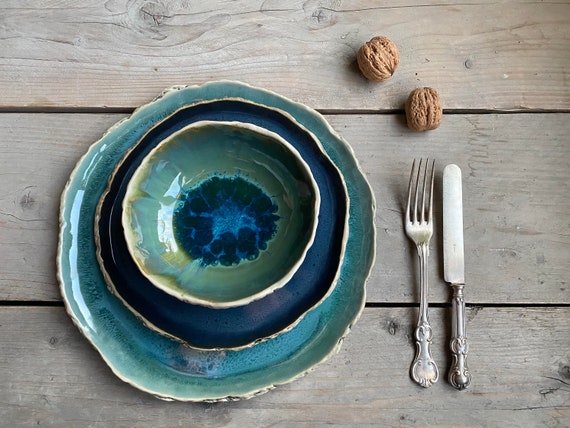This aerial color photograph captures a detailed, rustic table setting on a weathered wooden park bench table. The overhead perspective reveals the intricate grain of three individual wooden slats forming the tabletop. Central to the image are three ceramic stoneware pieces: a large turquoise plate at the bottom, a slightly smaller dark blue plate stacked on top, and a bowl with a green exterior and blue interior crowning the arrangement. The plates are handmade, evident from their slightly irregular shapes. To the right of this stack is an antique-looking silver fork and knife positioned upright, side by side. Just above the utensils sit two shelled walnuts, carefully placed, adding a natural element to the setting. The harmonious blend of teal, blue, and green hues with the rustic wooden background creates a visually captivating composition.